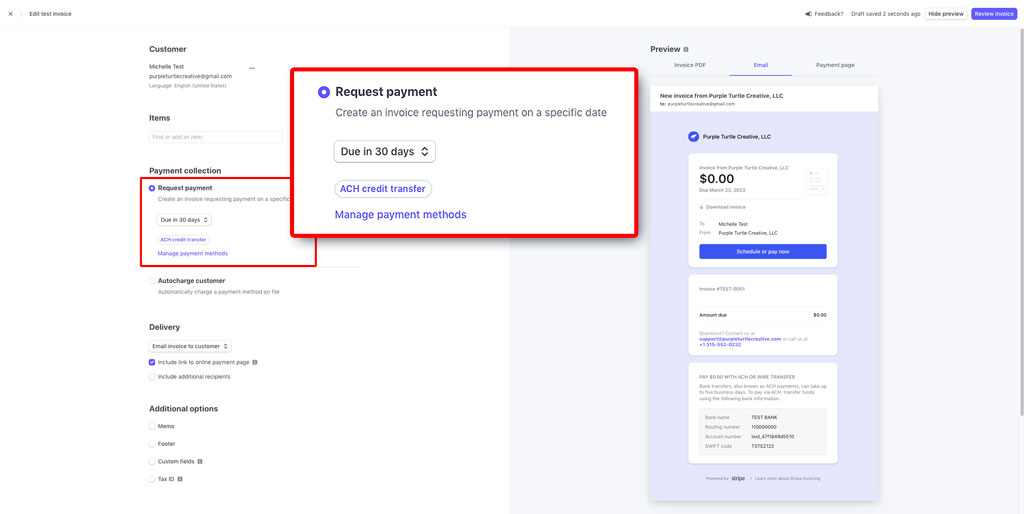This screenshot showcases a detailed section of a website interface, focusing on customer payment collection and delivery options. The text is notably small, making it challenging to decipher all the details.

In the top-left corner, "Customer" is prominently displayed, with additional smaller text underneath. Below this, the phrase "Payment Collection" is visible, with a red box enclosing the subsequent content, though the text within the box remains illegible due to its tiny font.

This section features a drop-down menu, followed by another labeled "Delivery," accompanied by three further lines of information. A set of options is available here, allowing the user to select one of two choices via radio buttons.

Below, under "Additional Options," four selectable bubbles are presented. 

On the right side of the screen, the word "Preview" is seen, presumably indicating how the content will appear on a mobile device.

Near the top, slightly off-centered to the left, another red-outlined box overlays part of the screen. Within this box, it instructs to "Request Payment," with the description, "Create an invoice requesting payment on a specific date." There's a drop-down menu for selecting the due date, currently showing "Due in 30 days" as an example.

Beneath this, a button labeled "ACH Credit Transfer" is situated, followed by a blue hyperlink that reads "Manage Payment Methods," suggesting further customization options for managing payments.